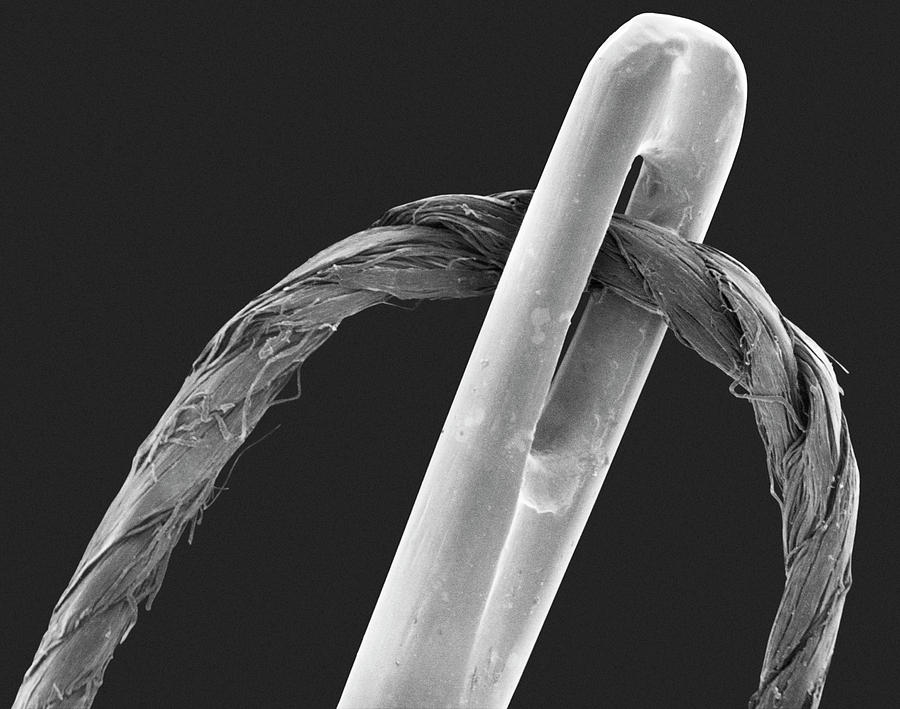This black-and-white photograph presents a highly magnified, extreme close-up image of a sewing needle and thread. The needle, appearing almost metallic and bright silver, contrasts starkly against the dark, black background. The focal point of the image is the eye of the needle—a large, elongated oval hole through which a piece of thread is threaded. The thread, depicted in intricate detail, displays a rough and fibrous texture, with individual fibers twisting together in a braided pattern and some unraveling at places. The needle projects from the center of the image, leaning slightly towards the right, while the thread enters from the bottom left, passes through the needle's eye, and then curves back down towards the bottom right. The entire composition emphasizes the incredible magnification, showcasing details on the thread and needle that are invisible to the naked eye, giving the needle an almost bone-like appearance and rendering the thread more rope-like in texture. The simplicity of the black backdrop further highlights the intricate details and texture of the needle and thread.